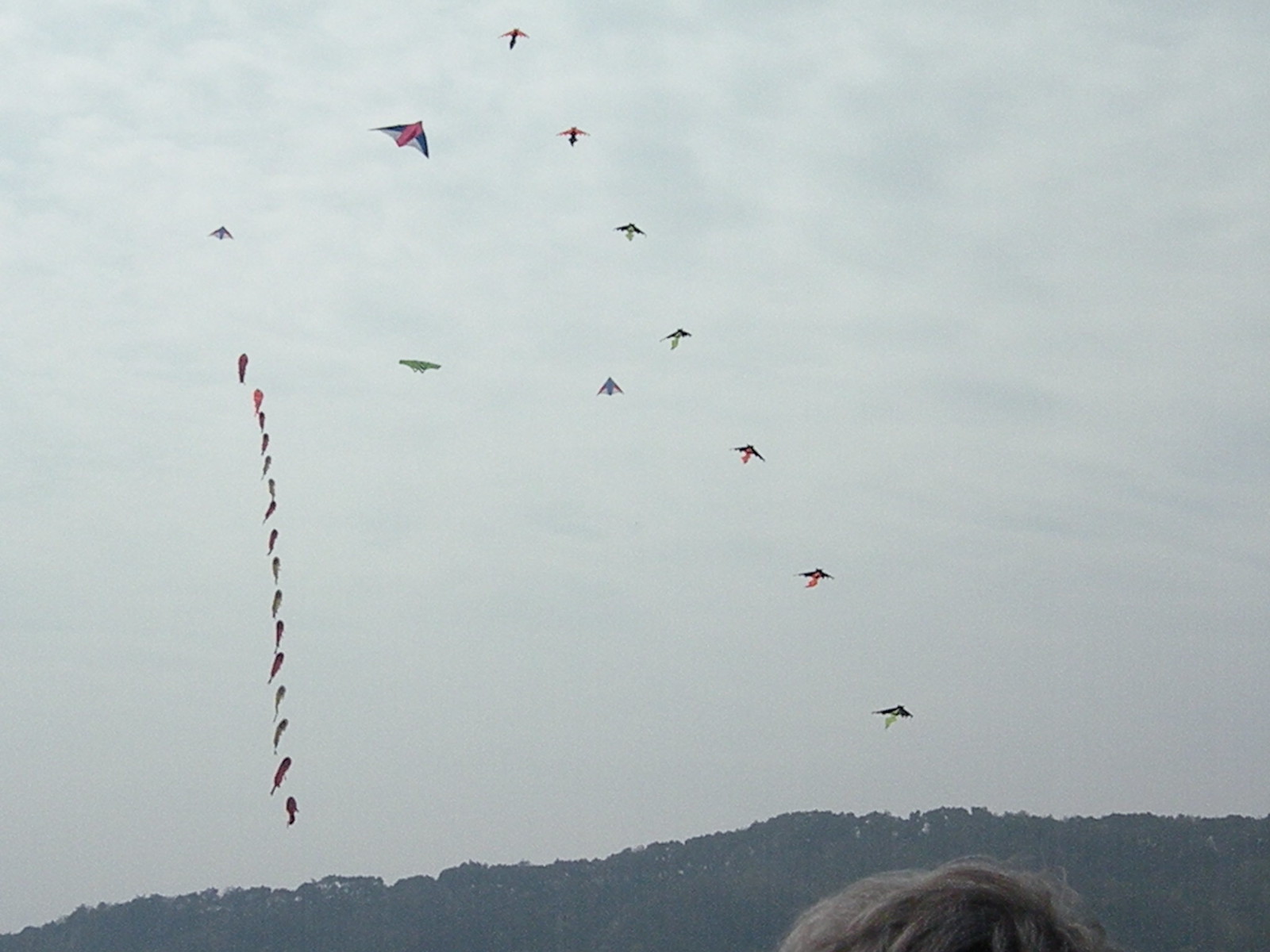This photograph, possibly AI-generated or taken with a long exposure, captures an overcast sky filled with an array of kites, implying a kite festival. The gray sky features scattered clouds, with a subtle brightness at the top indicating the sun's presence behind the clouds. The main focus is on the kites: a series of approximately 10 kites forming a straight diagonal line from the top to nearly the bottom of the image, and a vertical line of another 12 to 13 kites on the left side, resembling jellyfish with tentacle-like streamers. Some kites sport green or red streamers, adding splashes of color against the drab backdrop. At the very bottom of the photo, a tree line with a dense cluster of trees and shrubs is visible on a distant hill, and in the lower right corner, you can just see the top of someone's brown-haired head. This detailed and somewhat chaotic arrangement of kites, combined with the informal nature of the composition, gives a whimsical and spontaneous feel to the scene.